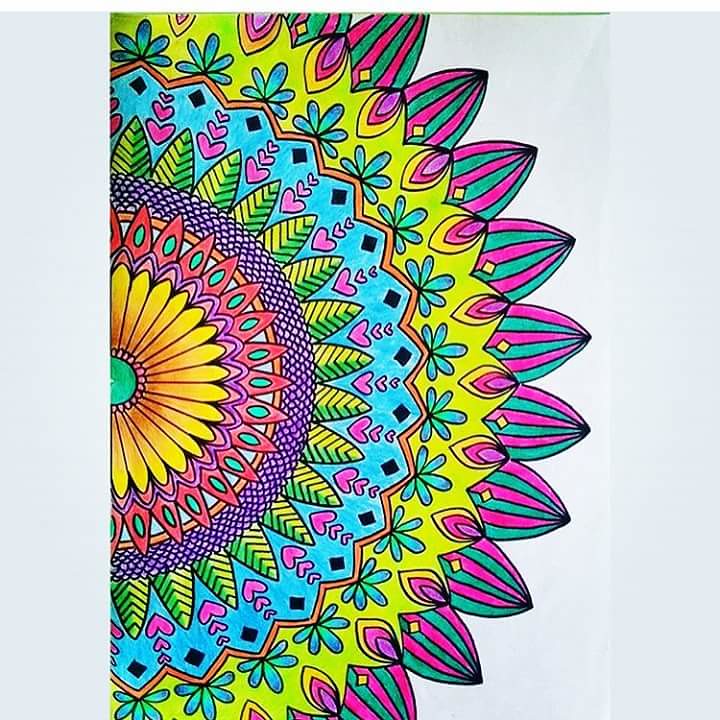The photograph captures an indoor, color image looking down at a piece of sketch paper that features a highly detailed geometric and floral pattern. The sketch appears to represent half of a radial design, reminiscent of intricate quilt patterns associated with Amish crafts or hex signs found on barns. The visible portion of the drawing is the right semicircle, with the upper and lower sections cut off.

The central focal point of the pattern is a yellow flower with approximately 16 thin petals encircling a green center. Surrounding this are various concentric rings of design with distinct colors and intricate details. The first ring includes light red elements followed by a band of light purple with a snake-skin-like texture. Next, blue leaves radiate outward, bordered by a series of small purple hearts.

An outer yellow band encircles these elements, followed by another layer featuring vertically striped leaves in purple and green. The entire design is filled with color, showing no exposed white areas, and the paper exhibits slight crinkling on the right side. In sum, the drawing is a vibrant and detailed representation of concentric geometric floral patterns, marked by its rich use of colors and intricate shapes.